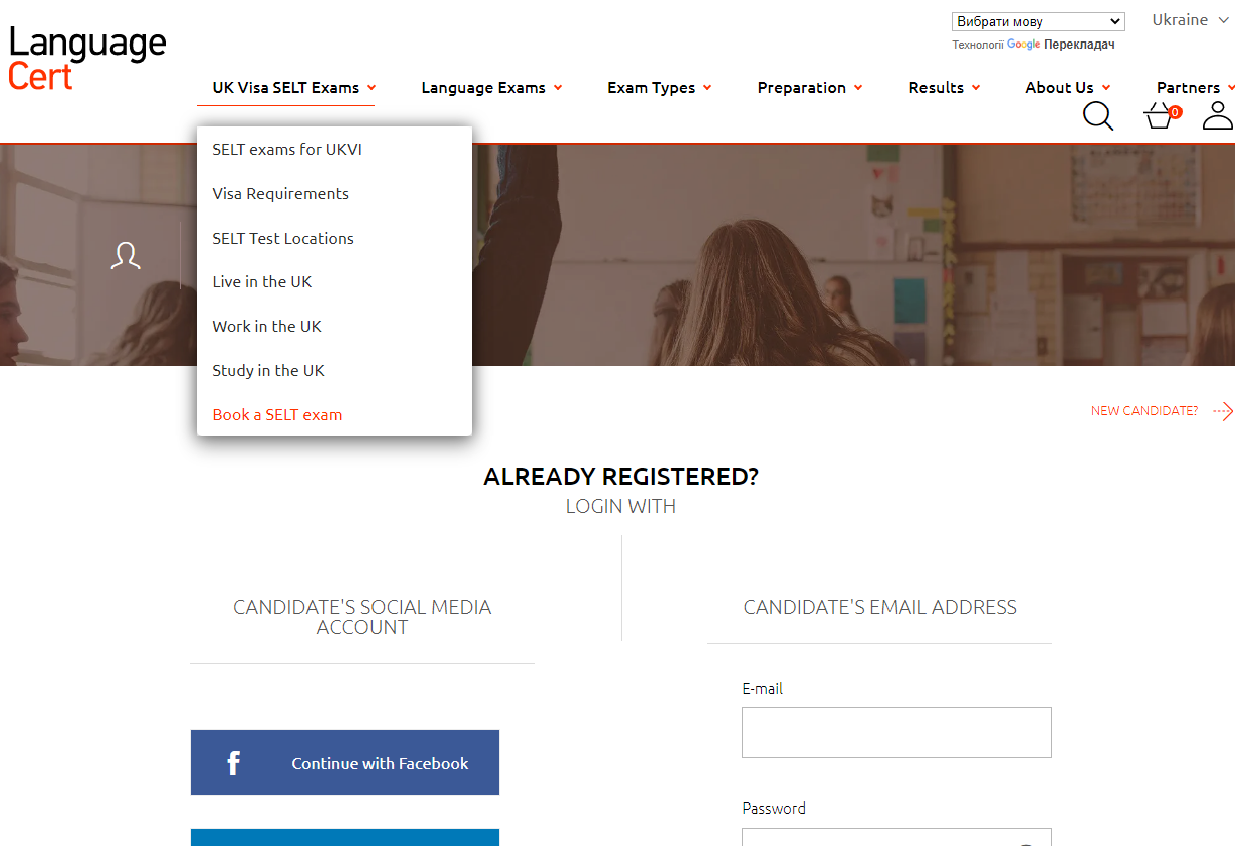Screenshot of a website's landing page for Language Cert. The page prominently features options for various examinations, including a UK Visa self-exam, indicated by a dropdown menu with an orange arrow. Navigation options include "Language Exam Preparation," "Results," "About Us," and "Partners." A central image shows a classroom setting. Beneath the image, there is a section for registered candidates to log in using their social media accounts or with their email and password. An orange link with a right-pointing arrow provides a registration option for new candidates. A clickable Facebook link is also available for pre-registration.